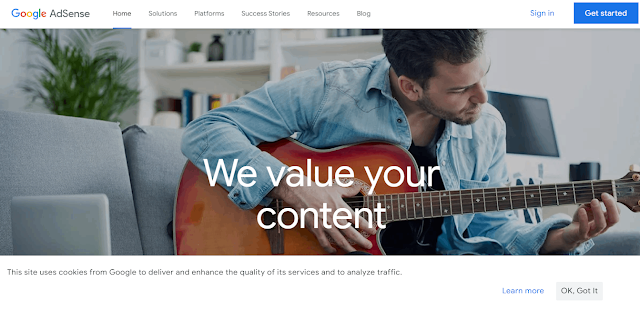The image depicts the Google AdSense sign-on page. At the top of the page, the header prominently displays "Google AdSense," with navigation tabs for Home, Solutions, Platforms, Success Stories, Resources, and Blog. On the right side of the header, there is a sign-in option accompanied by a bright blue "Get Started" button.

Below the navigation tabs, the main section features a large, captivating photo of a young man seated on a light gray sofa. The man, dressed in a blue denim shirt over a black undershirt, is playing a vibrant red guitar with brown strings. Overlaying the guitar, text reads, "We Value Your Content."

The scene is set in a cozy living space, where to the left of the sofa, a computer screen is visible. The man himself has short dark hair and is clean-shaven with a light beard. Behind him is a well-stocked bookcase containing decorative jars, books, and a green plant, adding a touch of natural decor directly behind the sofa.